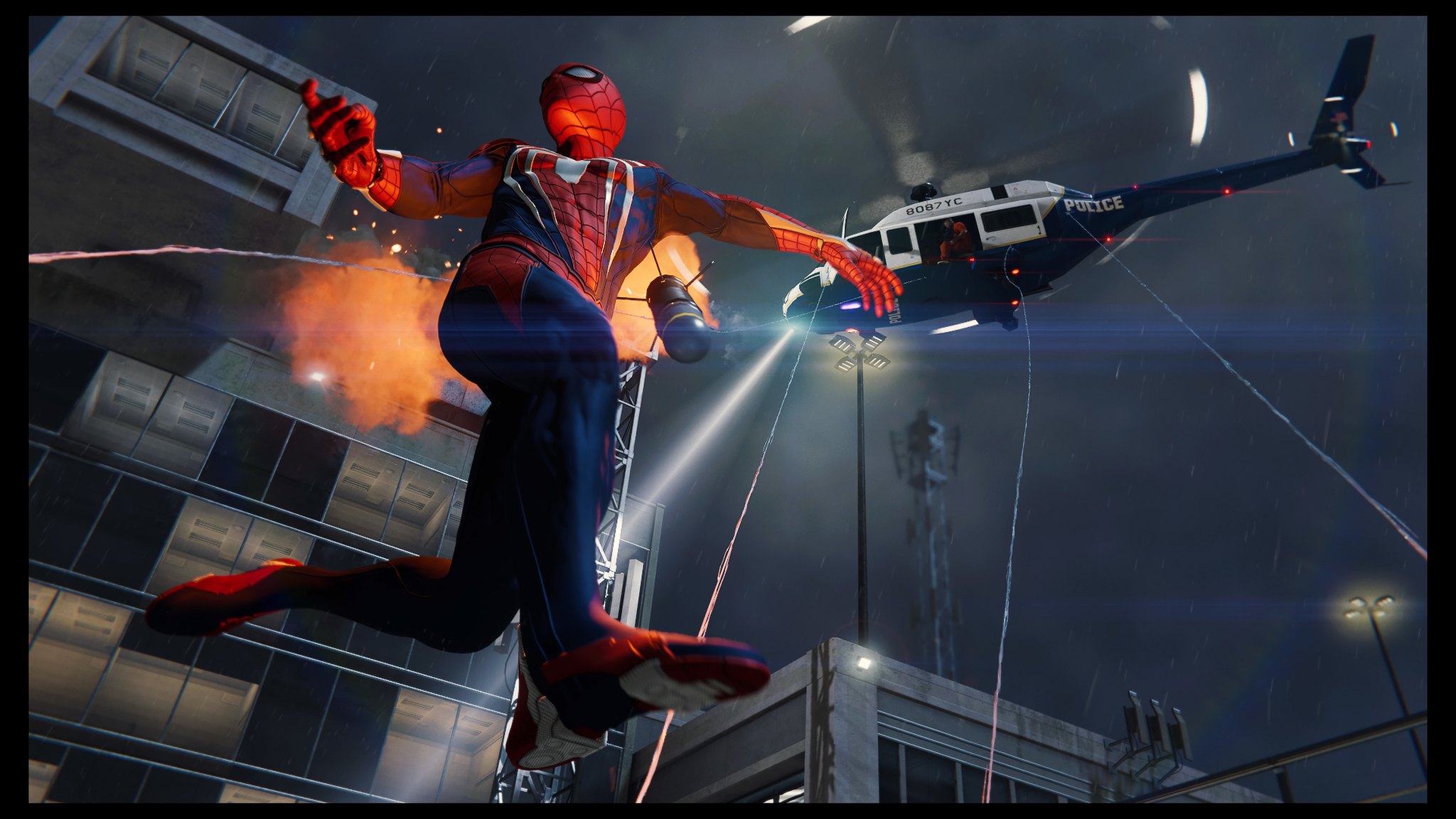In a dynamic and electrifying scene from a digitally animated Spider-Man universe, the viewer's perspective is angled upwards, capturing the thrilling airborne action. On the left, Spider-Man is mid-leap, twisting his agile body towards the right. His right leg is fully extended downward, revealing the red sole of his foot, while his left leg is bent at a 90-degree angle, with his foot flicked behind him. Spider-Man's left arm stretches forward with his hand pointing down, and his right arm is bent at the elbow, with the back of his knuckles facing downward, creating a dramatic pose. His head is turned to the left, intently focused on the action unfolding around him.

To the right of Spider-Man, a police helicopter hovers with its side door open and rotor blades blurred in motion, represented by a whirring circumference of highlights. A beam of white light from the helicopter's searchlight cuts through the scene, widening as it descends and partly illuminating a scaffold structure behind Spider-Man.

Adding to the intensity, an explosion erupts behind Spider-Man, with orange flames bursting out from beneath his left arm and behind his torso, casting a fiery glow. The backdrop features a towering office block type skyscraper on the left side of the image, with some windows appearing blacked out, others made of glass, and a few reflecting the orange hue from the explosion, suggesting either internal lighting or external reflection.

Spider-Man's iconic webs can be seen trailing from the police helicopter to various points in the background, weaving through the chaotic scene. The high-contrast elements, from the intense explosion to the detailed rendering of the helicopter and building, create a visually compelling and action-packed image that captures the essence of Spider-Man's thrilling escapades.